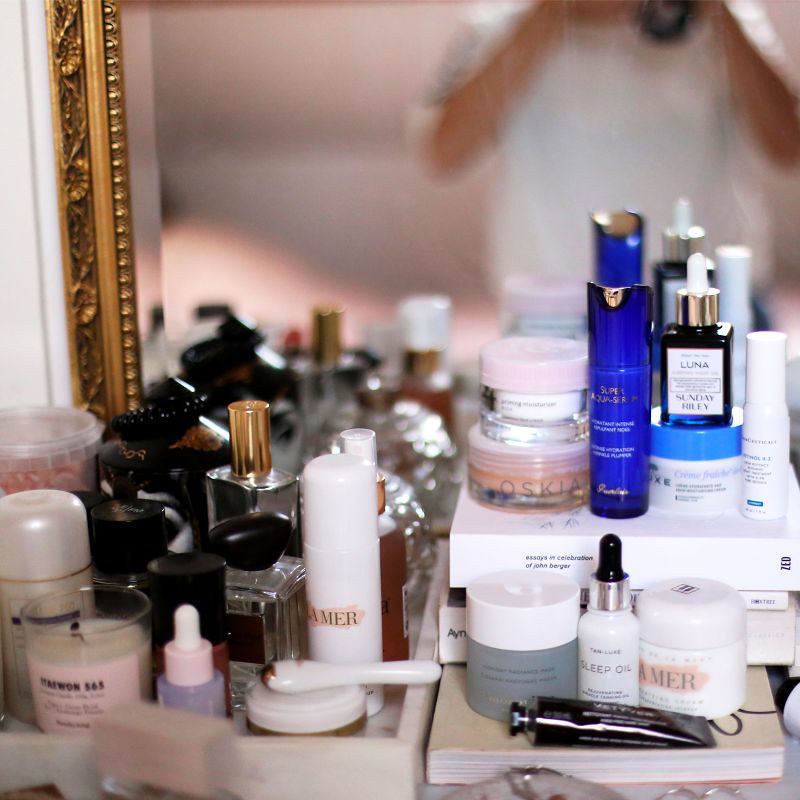This photograph captures a meticulously arranged lady's vanity table. Dominating the scene is an ornate mirror with a striking gold gilt frame. The frame features a bauble design closest to the mirror, transitions into a plain strip, and ends with an intricate old-fashioned floral and swirl pattern along its outer edge. The mirror itself is cut at an angle along the periphery, where it meets the frame, adding a touch of unique craftsmanship. Reflecting in the mirror, albeit out of focus, is the photographer, identifiable by their short-sleeve white top and the camera in hand, capturing the scene.

The vanity table is adorned with an array of feminine products. On the left half, a white box houses a collection of beauty items. Inside, there is a candle in a glass jar, several glass-bottled perfumes with black and gold lids, a small tub of product, a dropper bottle, and a spray bottle. To the right of this assortment lies a cream-colored book. Resting atop this book are a black tube containing a makeup product, two tubs — one featuring a transparent base and the other entirely white, as well as another dropper bottle. Further right, additional products are stacked on what appear to be more books or makeup boxes. Among these items is a vivid blue product, a few more skincare and cream tubs, and yet another dropper bottle, showcasing a rich collection of beauty and skincare essentials on this elegant vanity.